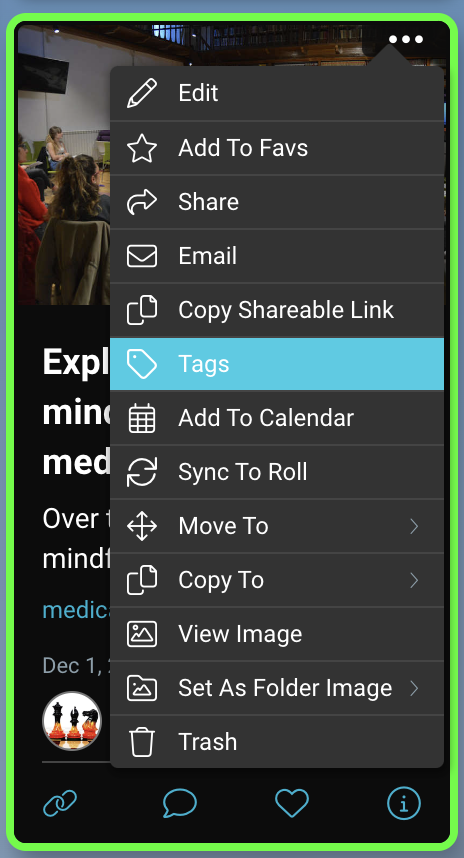The image appears to be a mock-up of a mobile phone interface. The mock-up is enclosed within a curved rectangle, set against a closely trimmed light blue background that enhances its prominence. At the top of the screen, partially visible and somewhat obscured by a large drop-down menu, there's an image that seems to depict people seated and listening to a speaker—though it's not entirely clear due to the truncation.

Below the obscured image, some partially visible text appears, likely labeled as "XPL," possibly short for "Explore," followed by "MIN" and "MED." The significance of these labels is unclear since the drop-down menu covers much of the content.

The drop-down menu itself is detailed with various icons accompanied by text, indicating different functionalities. The topmost option features a pencil icon labeled "Edit," followed by:

- A star with "Add to Faves"
- An arrow pointing back with "Share"
- An envelope marked "Email"
- Two overlapping pages indicating "Copy Shareable Link"
- A price tag icon marked "Tags" (selected and highlighted in blue, unlike the rest, which are gray)
- A calendar icon with "Add to Calendar"
- Two arrows forming a circle labeled "Sync to Roll"
- Four arrows pointing in all directions with "Move To"
- More pages marked "Copy To"
- A picture icon of a mountain and sun with "View Image"
- A folder containing the same image and the text "Set as Folder Image"
- A trash can icon labeled "Delete"

At the bottom of the screen, there is a navigation bar featuring icons for links, a speech bubble, a like button, and an information icon.

Overall, the image seems to illustrate a mobile application interface with a focus on organizational and sharing functionalities, though the full extent of its features is partially obscured by the large drop-down menu.